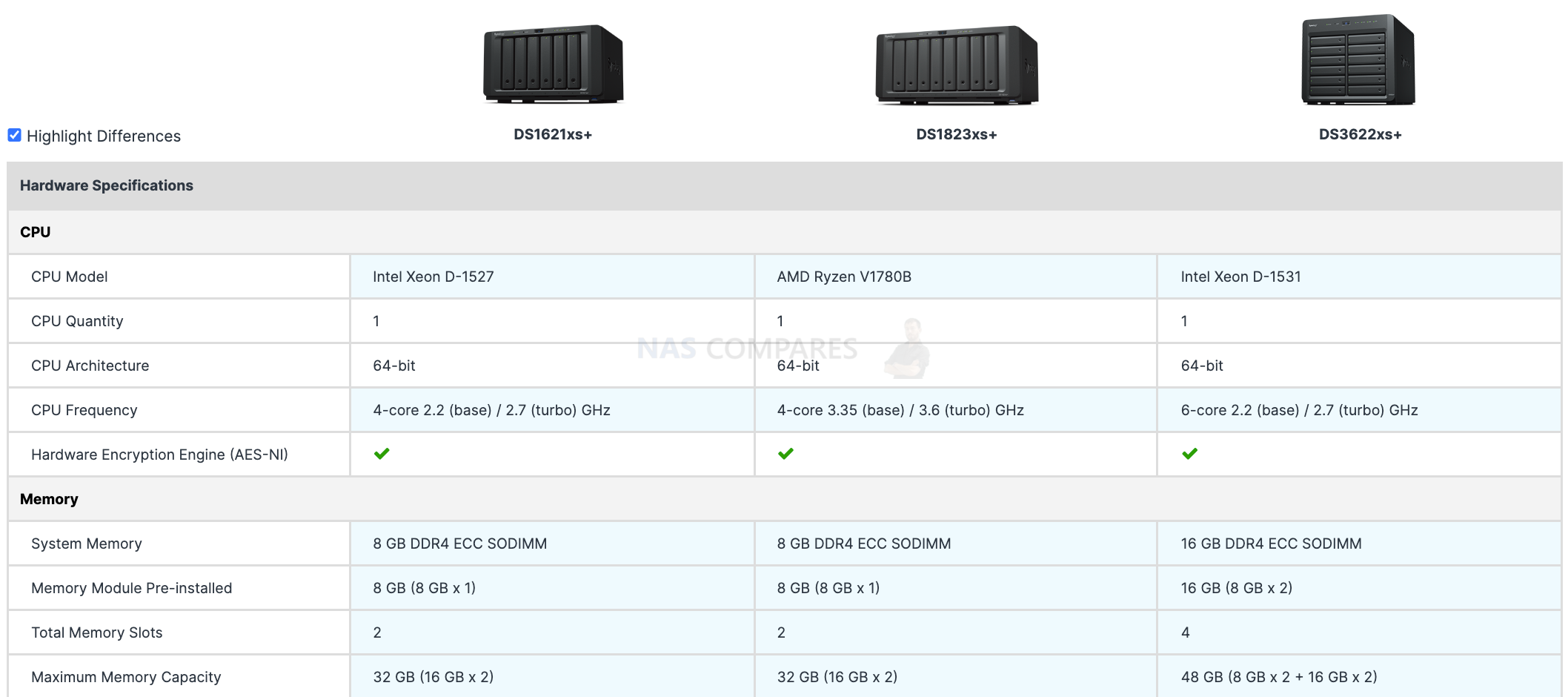A detailed comparison table showcases the hardware specifications of three different devices, namely the DS1621XS+, DS1823XS+, and DS3622XS+. Positioned at the top are images of these devices, which are essentially boxes housing various CPUs and memory components. The table below categorizes the hardware specifications into several sections.

The first section compares the central processing units (CPUs) of the devices, specifying the number of CPUs, CPU architecture, CPU frequency, and the presence of a hardware encryption engine. All three devices share a 64-bit CPU architecture and are equipped with a single CPU each, along with hardware encryption engines. 

Following this, a detailed breakdown of the system memory reveals that the DS1621XS+ and DS1823XS+ each come with 8 GB of pre-installed memory, whereas the DS3622XS+ is outfitted with 16 GB of system memory. Additionally, the table lists the number of memory slots available and the maximum memory capacity for each device.

Despite similarities in architectural design and encryption capabilities, the devices significantly differ in their memory configurations, providing a comprehensive overview of their respective hardware capabilities.